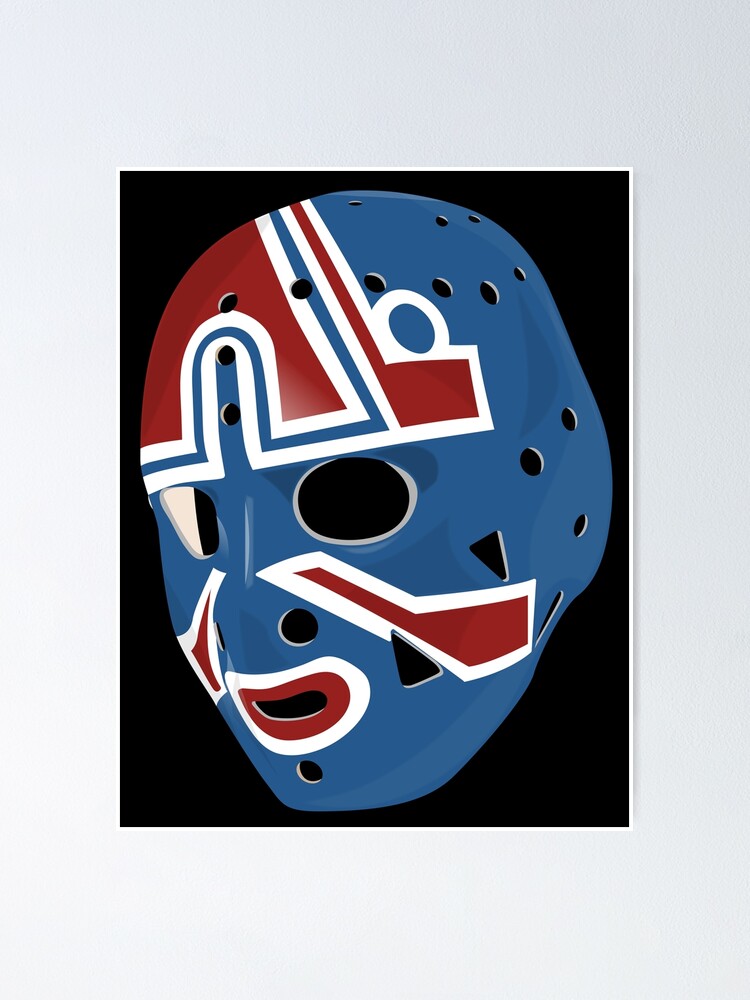This detailed image showcases a highly precise and meticulously detailed digital rendering of a full-face hockey mask against a solid black background. The mask, perfectly molded to fit over the entire face, including the ears, is predominantly blue and adorned with intricate red, white, and blue designs. A vivid red circle surrounds the mouth opening, which is further encircled by a white border. The mouth section also comprises a small, round breathing hole, appearing black due to the background, along with a slit for the mouth. 

A notable feature includes the red and white striped designs on the cheeks, and there's a prominent red 'A' on the forehead with a blue outline, followed by another white outline. Two hockey stick designs curve above the corners of the mouth, one towards the left cheek and the other above the right, enhancing the mask’s sports-themed decoration. The eye holes are regular-sized, and there are additional openings for the nostrils and chin. 

Subtle areas of shine enhance the mask’s realism, with notable highlighted spots on the bridge of the nose and near the left part of the mouth. This rectangular image is bordered by a thin white frame, beyond which lies a textured light blue background, emphasizing the vivid and striking colors of the mask. The overall depiction is a striking blend of artistry and attention to detail, capturing the essence of the sport and the intensity of the player behind the mask.